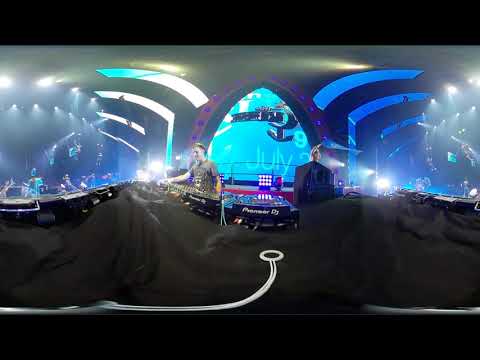In this fisheye, VR-style image, we see a DJ, identifiable by his green short-sleeved collared shirt, passionately controlling the audio at a club-like event. The DJ stands at a soundboard surrounded by numerous small, indistinct objects scattered on dark tables in front of him, with additional tables lining both sides of an aisle. The ambiance suggests a nightclub, emphasized by fluorescent lighting and a distorted turquoise center background screen displaying white text that reads "July 9". The image features distinct black bars at the top and bottom, adding to its unique visual framing. The setting appears active, with people seated at the tables on either side, partially illuminated by glaring overhead lights, hinting at an ongoing lively event.